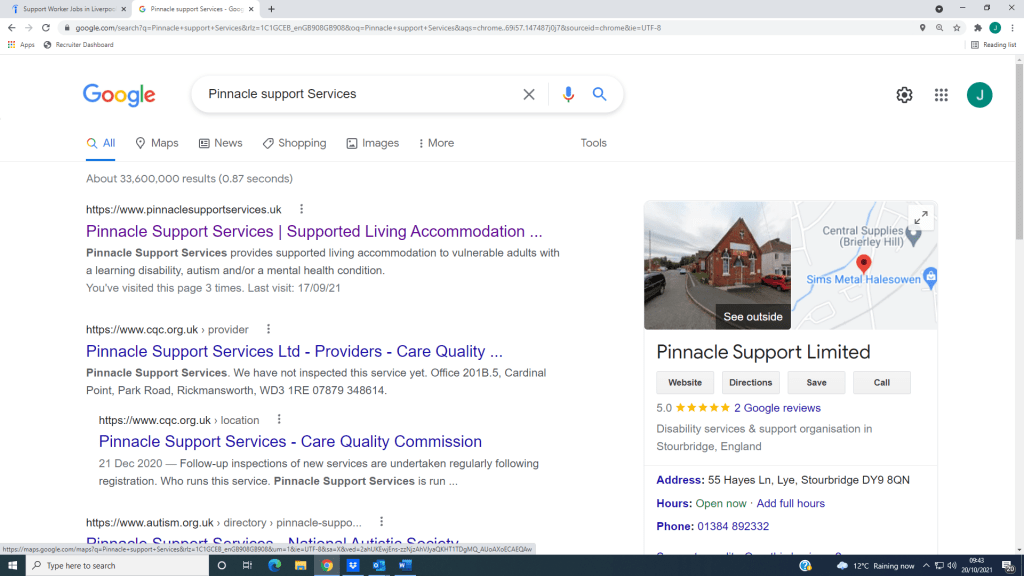The image depicts a search result page from Google for "Pinnacle Support Services." The search page features a horizontal navigation bar just below the search query, with the options "All," "Maps," "News," "Shopping," "Images," and "More." The word "All" is highlighted in blue, indicating the current selection, while the other options are gray.

The top search result, highlighted in purple to signify a previously clicked link, reads "Pinnacle Support Services - Supported Living Accommodations." Beneath this, subsequent entries include "Pinnacle Support Services LTD - Providers Care Quality" and "Pinnacle Support Services - Care Quality Commission." Additionally, part of another result is visible, reading "Pinnacle Support Services - National Autistic Society."

On the right-hand side of the page, there's an information panel for Pinnacle Support Services. This panel includes a photo tagged "See outside," a map displaying the location, Google reviews, the complete address, and a note in green indicating that the service is "Open now."